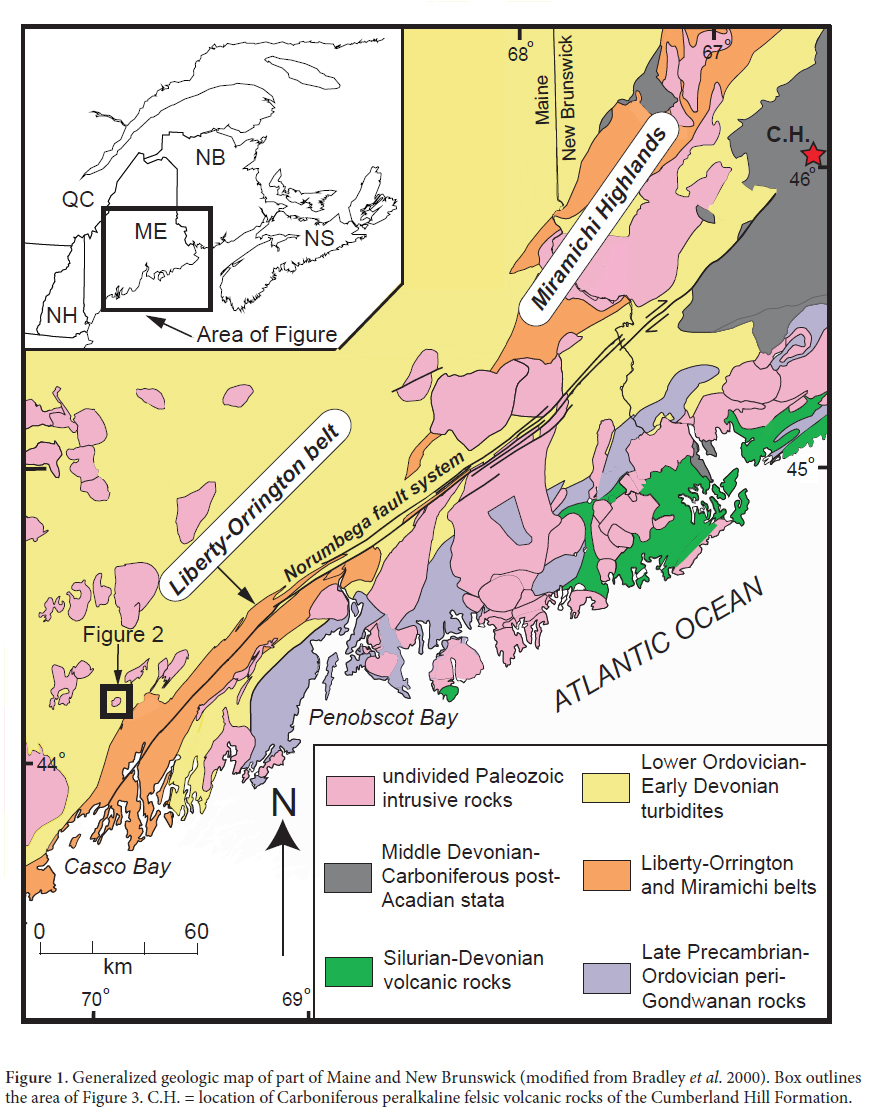This detailed map depicts the colorful geographic region along the Atlantic coastline of Maine and New Brunswick. The map highlights Penobscot Bay and is color-coded to illustrate various types of rocks, with distinct areas marked in yellow, orange, pink, green, and purple. These colors demarcate different geological features, such as undivided Paleozoic intrusive rocks in pink and Middle Devonian Carboniferous post-Acadian strata in black. The Atlantic Ocean is uniquely shown in white, standing out against the vibrant land areas.

An inset in the top left corner provides context, displaying the location of this section within the larger area of Maine, with a black and white square and an arrow indicating the specific area detailed in the main map. Key labels, such as the Liberty-Orington Belt and Marishee Highlands, are noted within the map itself.

A comprehensive key located in the right corner deciphers the coloring, and a scale in the left corner measures distances from 0 to 60 kilometers. Additionally, an arrow pointing north, labeled "N" in black, provides orientation. At the bottom of the map, a caption reads, "Figure 1 Generalized Geographic Map of Part of Maine and New Brunswick, Modified from Bradley et al. 2000," specifying that the box outlines the area of Figure 3, with "PH" marking the locations of Carboniferous, Percalinine, Felsic, Volcanic rocks of the Cumberland Hill Formation.